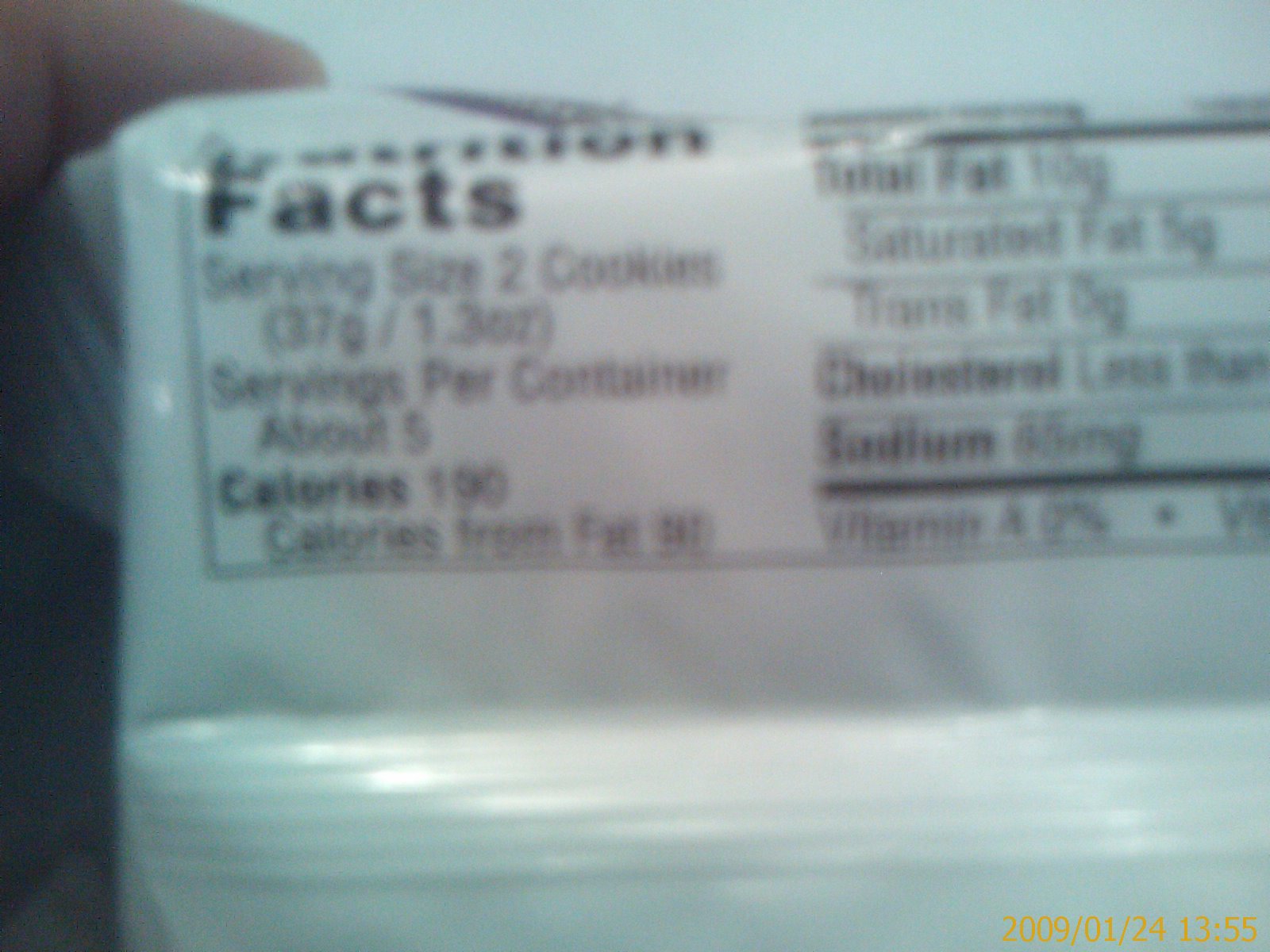This is a very blurry photograph of a person holding up a piece of food in a white wrapper to the camera, showcasing the Nutrition Facts label on the back. The image quality is poor due to a dirty camera lens, making the text hard to decipher. Despite the blurriness, the label indicates that the serving size is 2 cookies, weighing 37 grams or 1.3 ounces, with about 5 servings per container. Each serving contains 190 calories, with 30 calories from fat. The total fat content is 10 grams, including 5 grams of saturated fat and 0 grams of trans fat. Additionally, the label mentions cholesterol and sodium levels, which are unreadable. At the bottom right corner of the wrapper, there is a date in yellow text—January 24, 2009—along with a timestamp, though the exact details are difficult to make out due to the poor image quality. The reflection of the flash or ambient lighting further disrupts the clarity of the photograph.